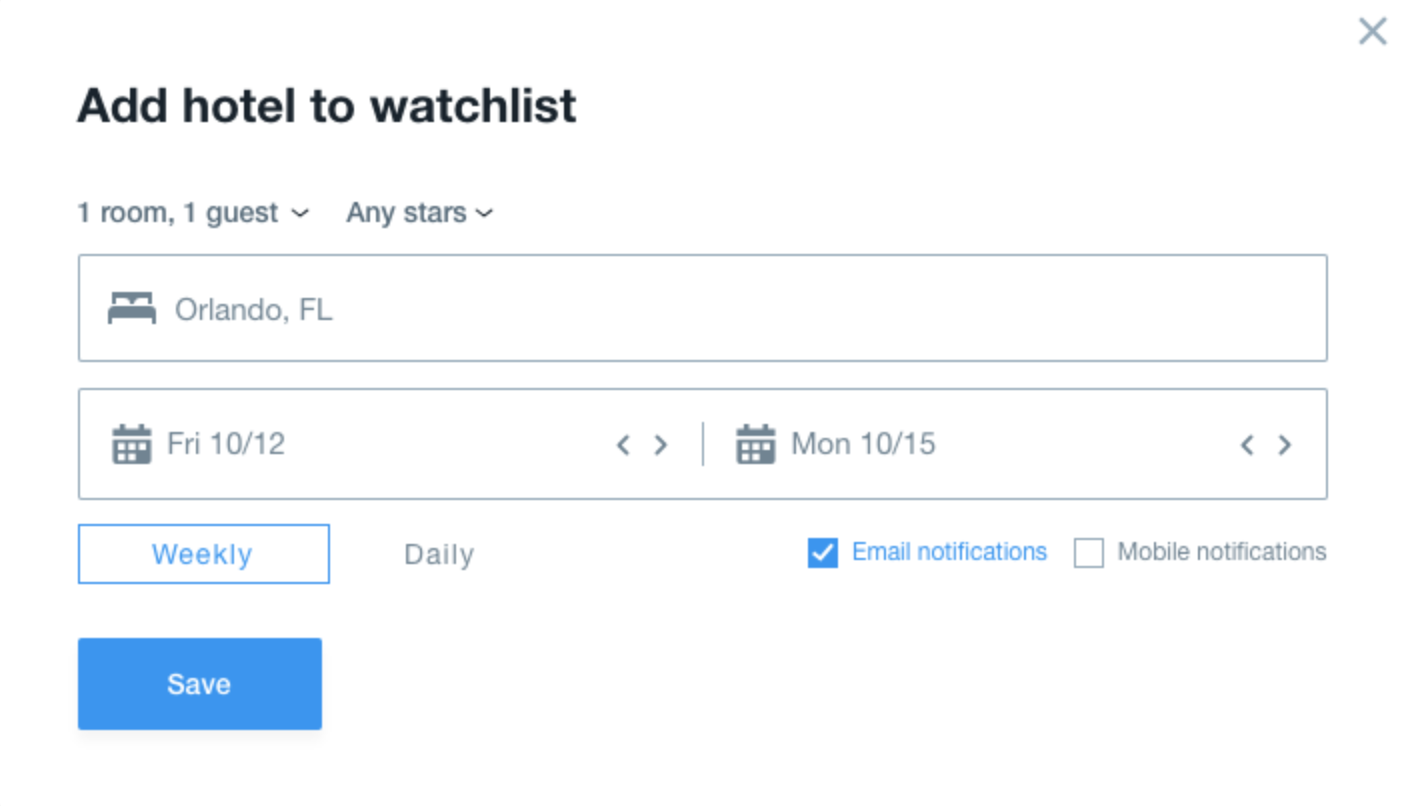This image showcases a hotel booking website interface specifically designed for adding a hotel to a user's watch list. The page indicates that a user has searched for hotel availability based on specific criteria: one room for one guest, with no specific star rating requirement, in Orlando, Florida. The booking dates selected span from Friday, October 12th to Monday, October 15th. Additionally, the user has opted for weekly email notifications about this listing. A prominent "Save" button is situated at the bottom of the screen, allowing the user to add the hotel to their watch list. Notably, there is no branding or identifiable information present to indicate which platform or hotel booking website this is. The interface appears as a streamlined dialog box dedicated solely to managing the watch list feature.